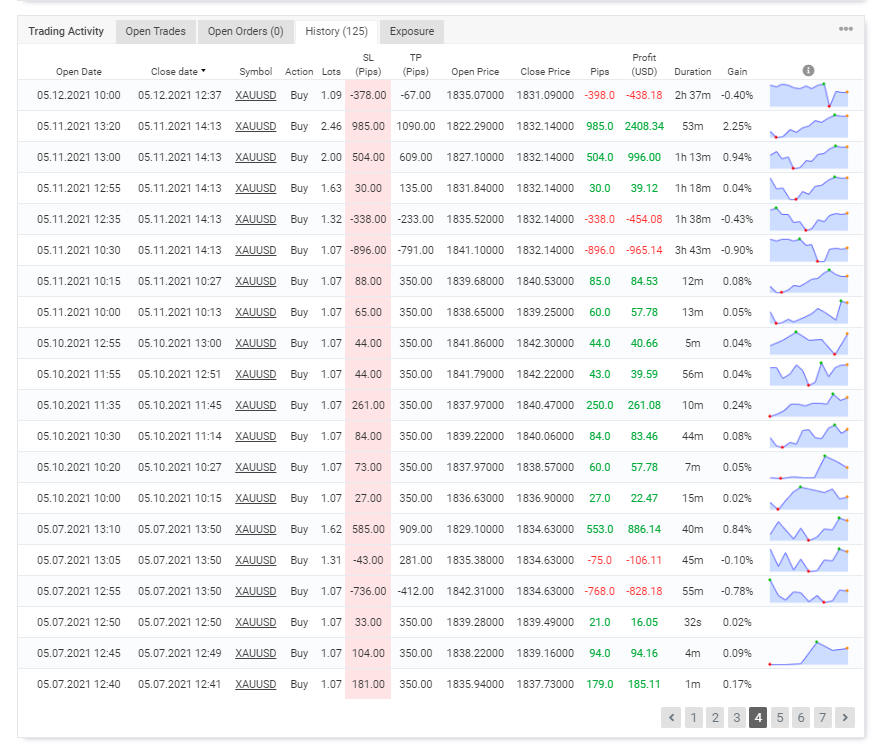The image showcases a comprehensive digital dashboard detailing stock trading activity, encompassing a wide array of stock tickers and their corresponding data. The interface features five selectable tabs at the top, namely: "Trading Activity," "Open Trades," "Open Orders," "History," and "Exposure," offering users diverse views into various aspects of their trading portfolio. The central section of the screen is populated with numerous columns and rows of numerical data, representing different metrics and values relevant to the listed stocks. Notably, one of the columns, labeled "SL" followed by unreadable text in parentheses, is distinctly highlighted in red, indicating a significant or alert status that requires attention. Due to the resolution, the specific numbers and further textual details remain unclear, preventing more precise interpretation of the data.